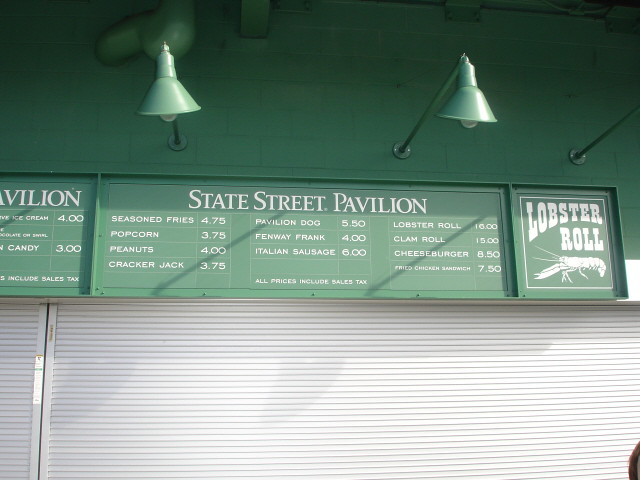This vibrant color photograph captures the front façade of a charming restaurant named "State Street Pavilion.” Dominating the upper half of the image, we see the side of the building which is painted in a lively shade of green. Two green lamps are mounted on the building, casting a gentle light that highlights the establishment's name prominently displayed in white letters – "State Street Pavilion." To the far right of this sign, the word "Lobster Roll" appears, also in white, accompanied by a small drawing of a lobster, hinting at the seafood delicacies awaiting inside.

Beneath the main sign, a secondary panel showcases some of the menu offerings, written in white text on the green background. The legible items include seasoned fries, popcorn, peanuts, Cracker Jack, Italian sausage, lobster roll, clam roll, cheeseburger, and Pavilion Dog, though a few items remain unreadable.

The bottom of the photograph reveals a steel metal gate, indicating that the establishment is currently closed. Bright light reflects off the gate, adding a touch of contrast to the overall scene. The detailed and colorful presentation invites curiosity about the restaurant's offerings and ambiance.